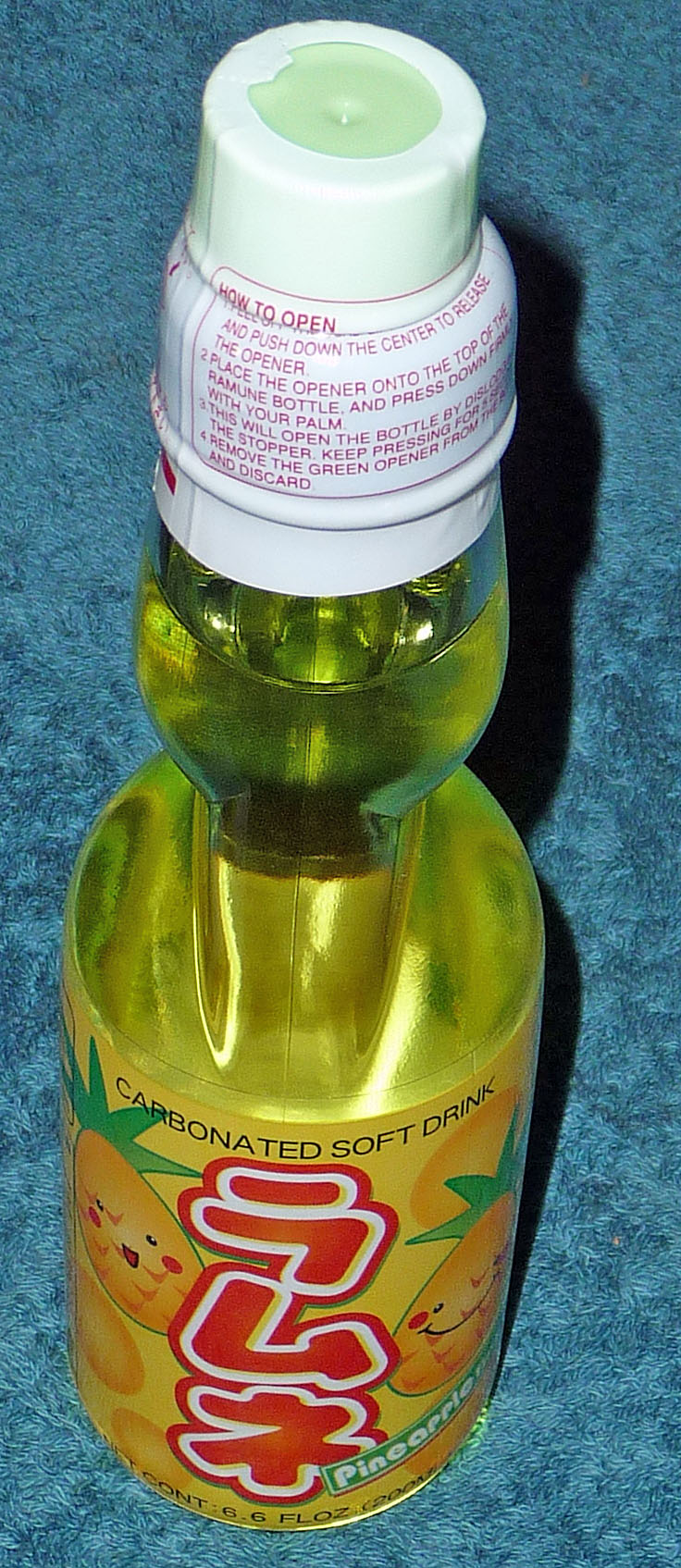This image captures a unique Japanese or Chinese carbonated soft drink displayed from a top-down perspective. The drink is housed in a distinctively small bottle featuring a round bottom that tapers dramatically to a narrow neck before slightly flaring out again at the smaller round top. The bottle is sealed with a white plastic cap wrapped in white plastic adorned with red text that provides instructions on how to open it. The liquid inside is yellowish in color, suggesting a fruity flavor.

An orange label wraps around the bottom round portion of the bottle, with the words "carbonated soft drink" prominently displayed. The label is adorned with whimsical illustrations of oranges on either side of the vertical Chinese characters in the middle. Additionally, on the bottom right corner of the label, there is an angled green rectangle containing the word "pineapple" written in white text.

This thoughtfully designed bottle combines playful aesthetics with functional details, making it an intriguing and attractive soft drink option.